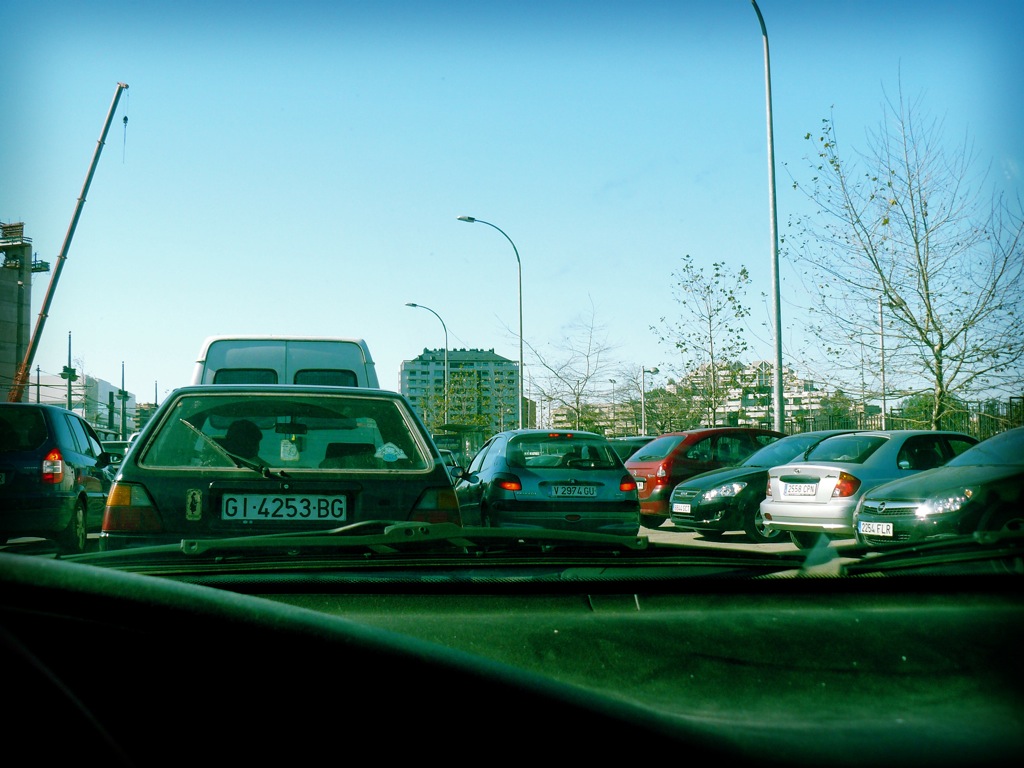A real-life photograph, taken from the interior of a vehicle moving down the road, captures a scene of heavy traffic with a distinct vintage feel. The interior features a black dashboard that curves up towards the steering wheel's rear, partly obscured in shadow with some visible dust. The windshield and black wipers frame the view of the congested road ahead. At the bottom center, the dashboard edges into the image.

Directly in front, a small, older hatchback sedan with the license plate "GI-4253-BG" appears, hinting at an unfamiliar country of origin. In front of this car, a white van, possibly used for transporting medical supplies, is visible. To the right, a black SUV and a silver minivan accompany this sedan, with more modern hatchbacks flanking the scene.

Parked along the right and diagonally from the image’s center are cars in a parking lot: a black car, a silver one, a dark green or black one, and a red one. The parking area is lined with gray lampposts and budding trees, their dark green, yellow, and brown hues indicating the season’s early growth. The sky above shows a clear blue with some white at the horizon.

In the distance, behind the static and moving vehicles, are an array of buildings, the tallest being white. A tall crane with a dark chocolate base transitioning to light gray reaches over on the left, its hook visible. This industrial touch underscores the setting's urban-industrial vibe, further enhanced by bare trees and the faint green hue enveloping the entire photograph, adding a nostalgic, almost filtered effect. The scene captures a bustling city moment frozen in time, marked by dense traffic and a distinct vintage ambiance.